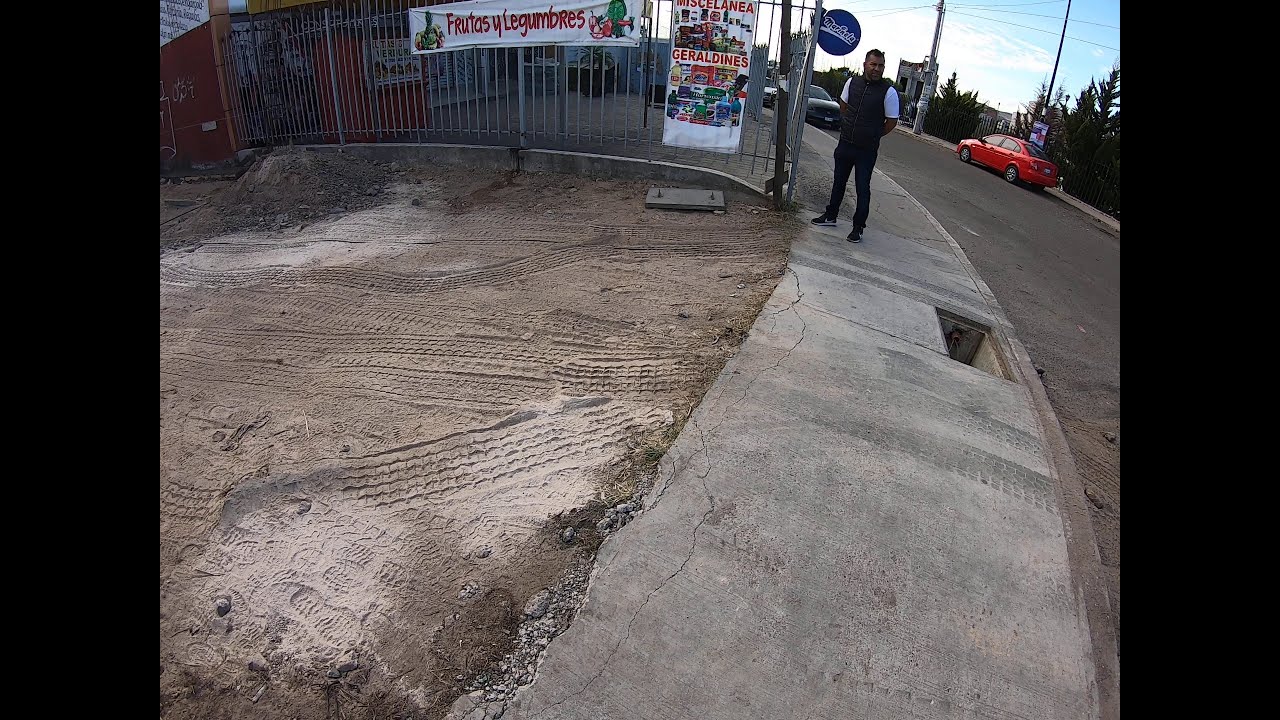The image depicts a man standing on a sidewalk beside a curved street, indicative of an outdoor, daytime setting that appears to be within an impoverished country. The man, characterized by his dark skin and black hair, is dressed in a white t-shirt underneath a black vest and pants, and is looking away from the camera. Behind him, a red car is parked along with several other vehicles on the street. 

The street scene is framed by a clear blue sky scattered with white clouds. Utility poles and lampposts line the street, complemented by some trees. Adjacent to the man, there's a sidewalk with an underground drain and a fence adorned with banners. One banner reads "Frutas y Legumbres," and another advertises "Miscellanea Geraldine's," both displaying images of fruits and various products. Behind this fence, there's a building that resembles a closed shop or restaurant. In front of the man lies an empty dirt lot marred with tire tracks and footpaths, suggesting infrequent use and neglect. The entire photograph captures the contrasting textures and colors, including red, black, white, gray, beige, brown, and silver, with the central focus on the man and the surrounding urban elements.